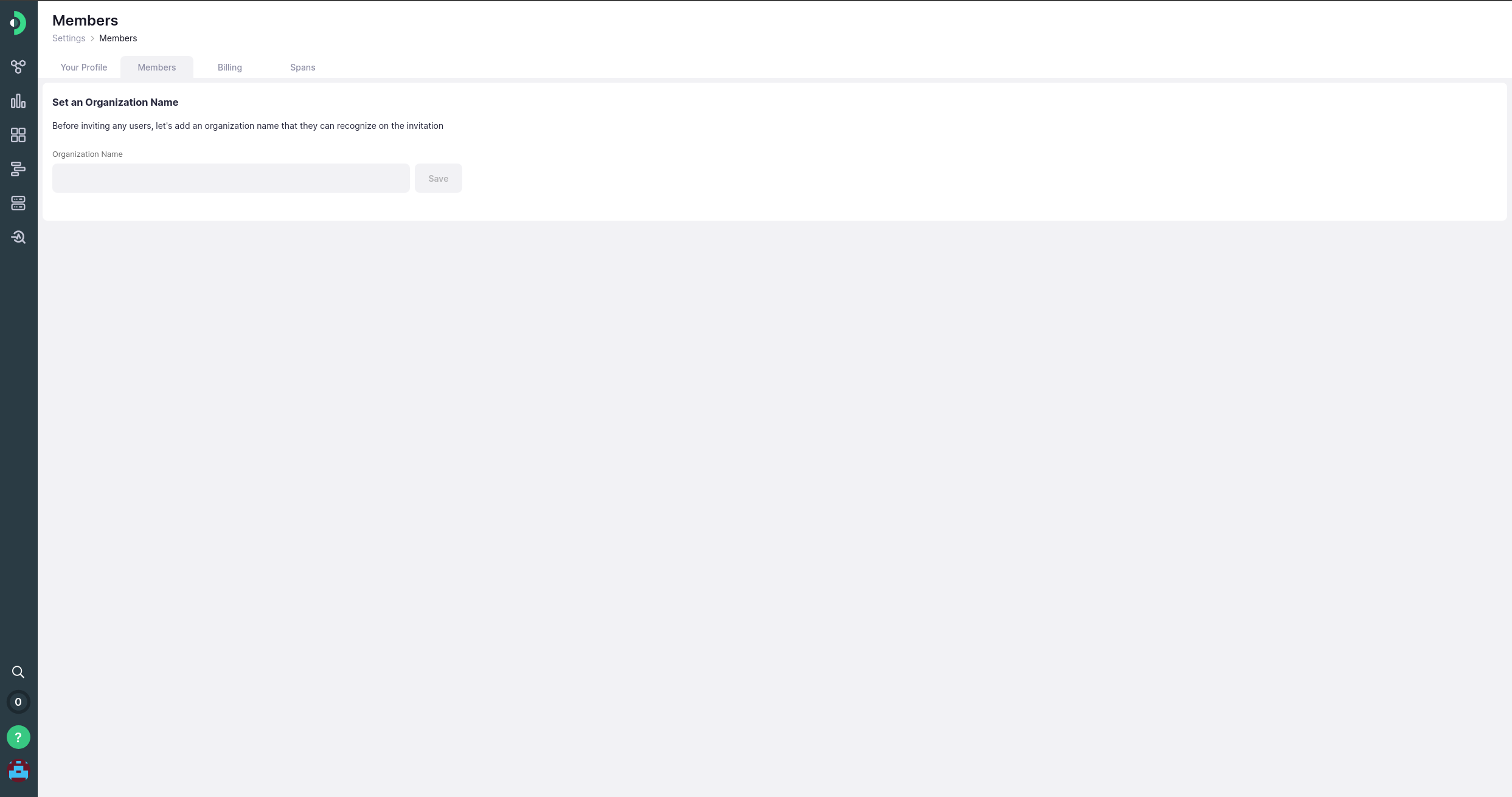In this image, we see a screenshot from a website or application with a clean, minimalistic design. At the very top left-hand corner, the header displays the word "Members" in black font. Below this header, there are four navigation tabs titled "Profile," "Members," "Billing," and another tab with text that is unreadable due to the image quality. This page appears to be designed for managing members within an organization.

On the left side of the page, a vertical black taskbar includes several icons representing different functionalities. These icons likely serve as shortcuts for editing content, searching within the site, and accessing a menu. The overall page background is white, providing a stark contrast to the black text and icons, which enhances readability. Despite the minimalistic design, the focus on member management is clear from the layout and available options.